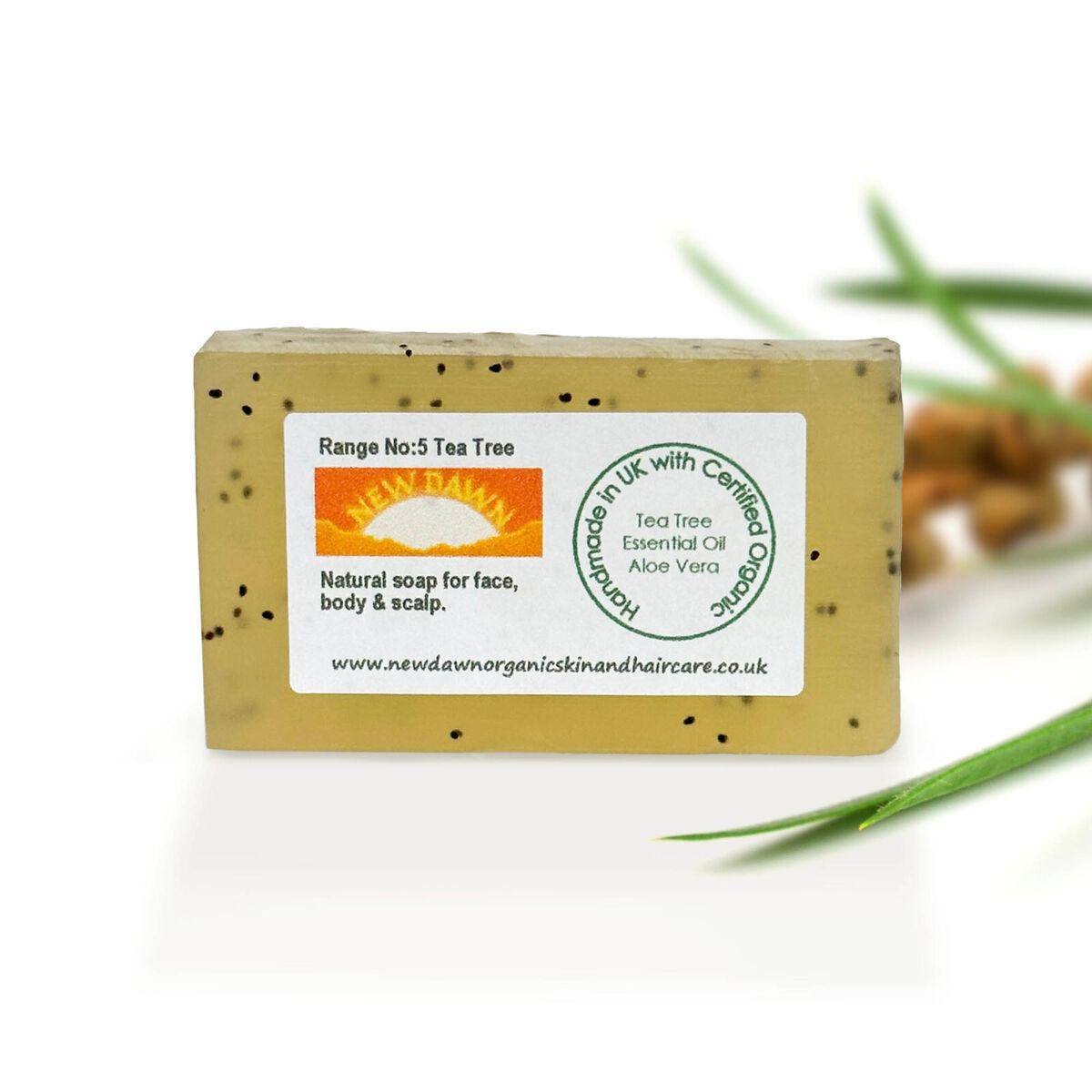The image features a handmade, natural soap bar prominently. The bar appears yellow with black specks resembling pepper grains. The label on the soap bar includes detailed text: "Range No. 5 Tea Tree" in black font, with "New Dawn" as the brand name, accompanied by their orange logo depicting a sun and clouds. This soap is specified for use on the face, body, and scalp. To the right, an out-of-focus area shows natural elements like branches and grass, emphasizing the soap's natural composition. A circular logo, printed in green, indicates that the soap is "Handmade in the UK with Certified Organic Tea Tree Essential Oil and Aloe Vera." The website www.newdawnorganicskinandhaircare.co.uk is also displayed on the label. The overall color scheme includes shades of yellow, green, orange, brown, and white.